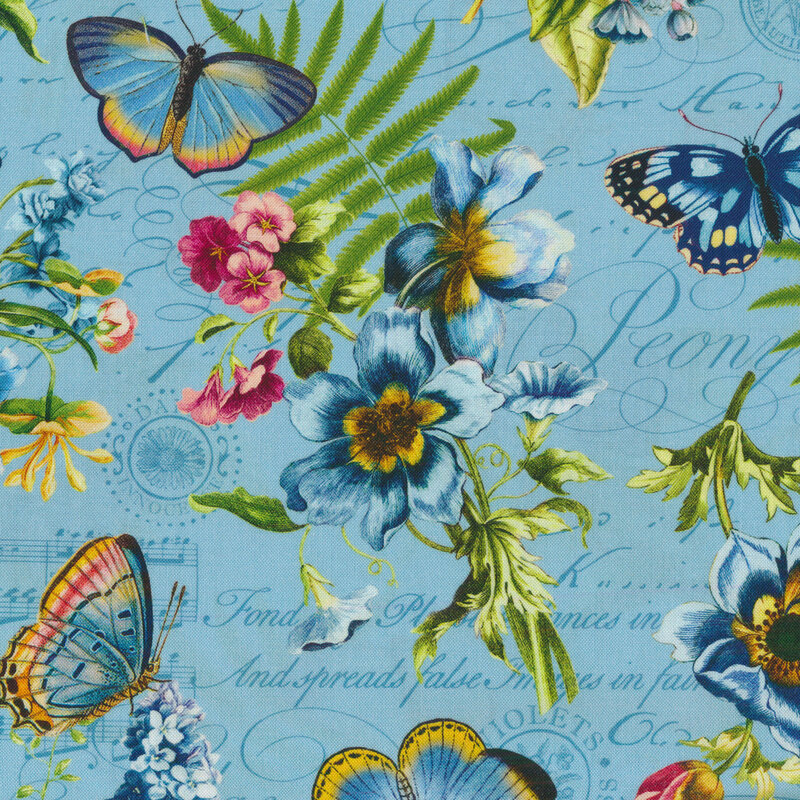The image features a richly detailed and vibrant blue background adorned with flowing cursive script that includes words like "peony" and phrases such as "fond and operates" and "and spreads false images in fair." Overlaying this backdrop is an intricate pattern of colorful butterflies, flowers, and leaves. The flowers vary in types and hues, featuring blue daisies with dark centers and yellow interiors, as well as pink flowers with gradients from darker to lighter pinks. Fern-like green leaves add to the foliage, and several butterflies with blue, yellow, orange, and red hues flutter around, many with striking blue wings tipped in yellow and red. Notably, a central blue flower has a distinct dark center surrounded by a yellow ring, and a delicate pink flower with smaller blooms appears nearby. The imagery is further enriched with subtle elements like postmarks and curly script that add a vintage, whimsical feel to the overall composition.